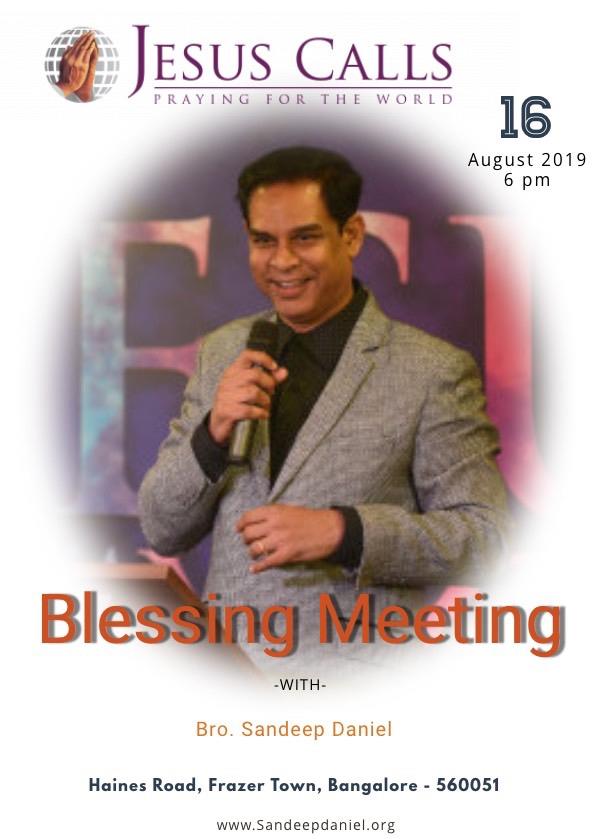In this photograph, a South Asian man, likely Indian, is standing on a stage, smiling and speaking into a black microphone. He is dressed in a gray blazer over a black shirt. The background features a large purple banner with white lettering partially visible, and the entire image is overlaid on a larger white background. The top of the image is marked with the text "Jesus Calls: Praying for the World," alongside a logo of a globe with clasped hands. Below this, it reads "16 August 2019, 6 p.m." Further down, the text "Blessing Meeting with Brother Sandeep Daniel" is displayed, followed by the location details: "Haynes Road, Fraser Town, Bangalore - 560051." Centrally at the bottom of the image is the website "www.sandeepdaniel.org."